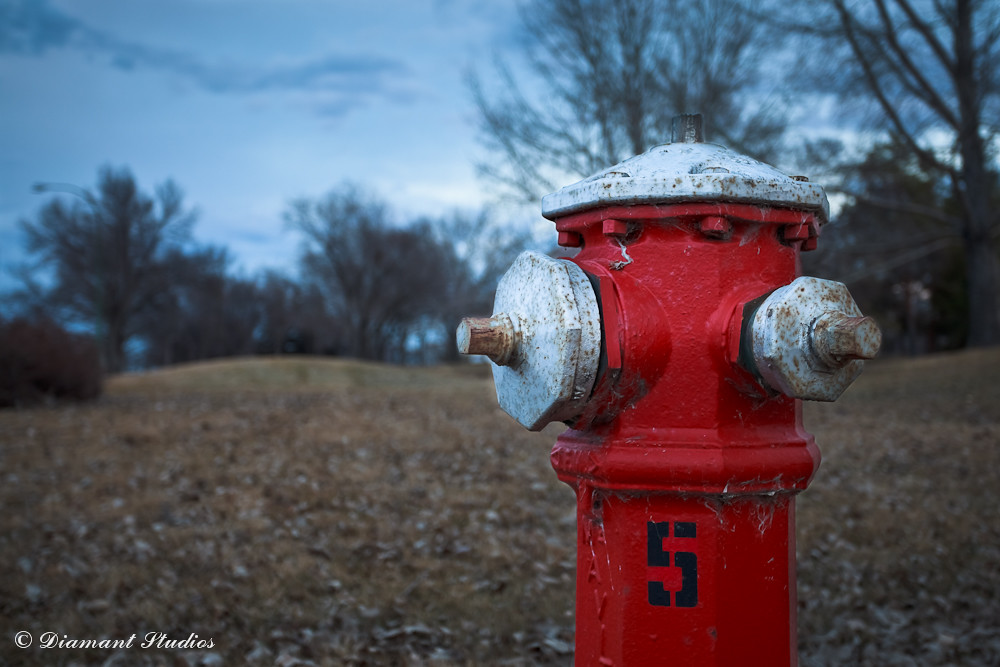The image features an old, weathered fire hydrant prominently placed in the foreground, presumably manufactured by Diamond Studios, as indicated by the copyright symbol "D-I-A-M-A-N-T" visible in the bottom left-hand corner. The hydrant stands 8 to 10 inches tall and is predominantly red, with three large white rust-covered knobs for hose connections on the top, right side, and left side. Its silver top is also noted. A bold black number "5" is painted on the front center of the hydrant. The background, though blurred due to the photo's focus on the hydrant, showcases a serene, outdoor scene with brown leafless trees and a beige-tinted grass field suggesting fall or early winter. The sky above is a darkened blue, contributing to the chilly atmosphere of the setting.